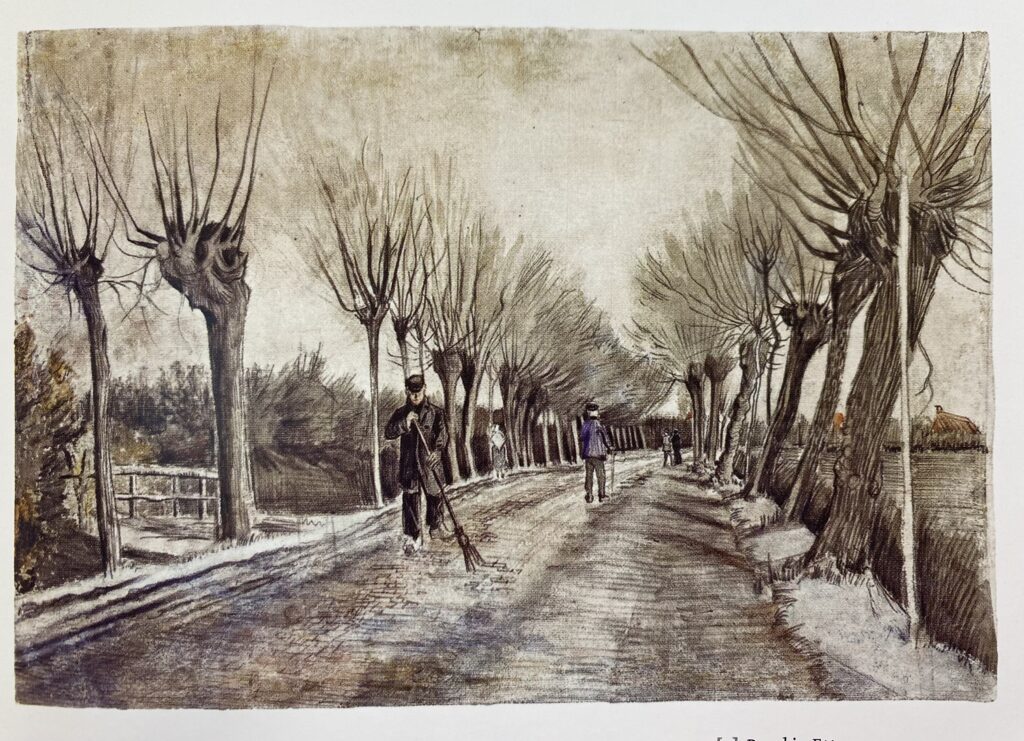The image is a scanned piece of artwork depicting a winter scene on a street and in a park area. In the foreground, there's a man sweeping a pathway; he wears a cap, which suggests he might work for the city, and is dressed in a black coat extending past his waist, black pants, and white shoes. An elderly man in a blue coat, black hat, and green pants, using a cane, is also seen walking on the path. Further back, two more figures are visible in the distance, bringing the total number of people to about four or five. The pathway, possibly the main street, is lined with peculiar, leafless trees that branch only at their tops. The trees on the right side of the path lean heavily to the right, while those on the left stand more vertically. Additionally, there is a field at the same elevation as the street on the right and a wooden fence located further left, below the street level. The scene is captured as if the camera is pointing down the street, offering an encompassing view of this serene yet somewhat desolate winter environment.